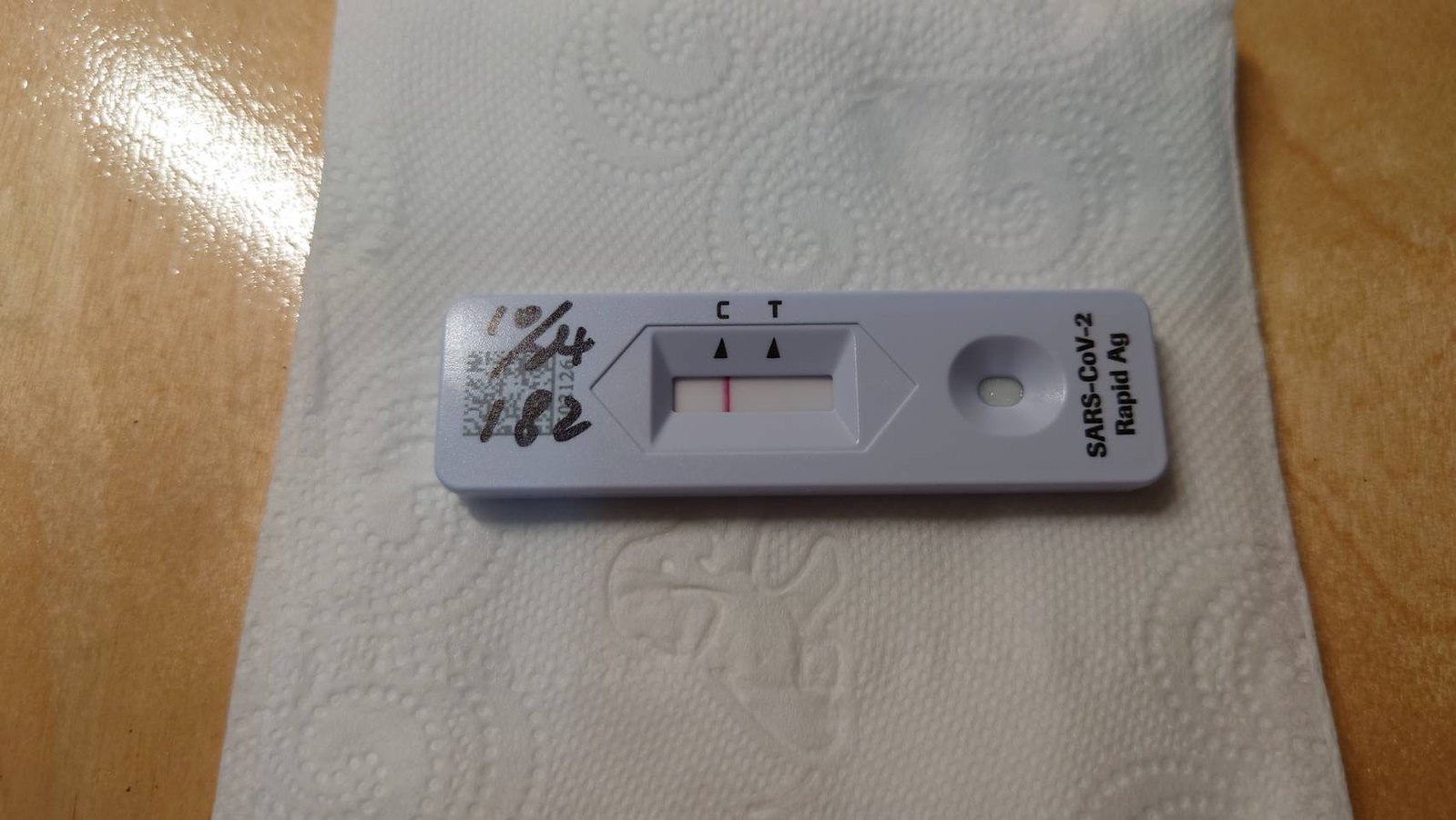This photograph features a COVID-19 rapid antigen test resting on a sheet of toilet paper that has a whimsical puppy pattern. Both the test and the toilet paper are white, creating a monochromatic backdrop. The test itself is marked with black lettering, including a "C" and a "T" at the top, with a noticeable notch cut out in the middle. Above this notch, there is a small round hole, and at one end of the test, the label reads "SARS-COV-2 RAPID AG" in black font. Along the bottom edge, a date is inscribed along with the number "182," sitting just above a QR code. The testing surface shows signs of being marked with a Sharpie. Notably, in the middle notch, there is a small white window displaying a red line under the "C," indicating the control line, while no line is visible under the "T," suggesting a negative result. The scene is set on a table with a warm, blonde wood finish.